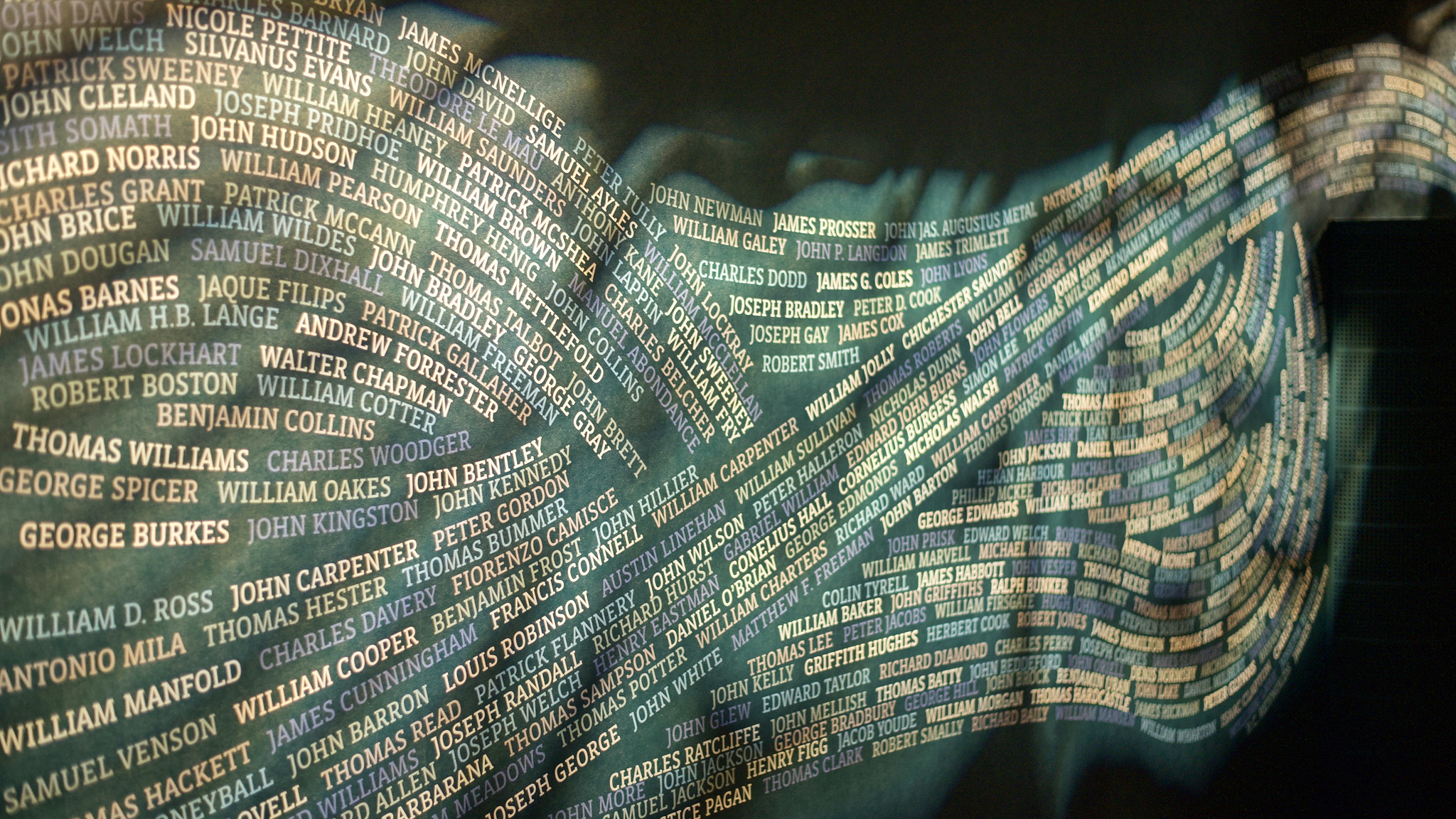In this horizontal rectangular image, the background is a solid black, creating a stark contrast to the vibrant shapes and names displayed prominently. The central shape starts as a rounded form on the left and narrows toward the right, fading into the upper right corner of the image. This form is adorned with a spectrum of colors, including greens, whites, yellows, grays, and various shades of teal and aqua. The most striking feature is the multitude of men's names imprinted across this shape, some in white, some in light blue or aqua, and others in yellow or light hues of red. The names, such as John Hudson, Richard Norris, William Pearson, Thomas Nettlefold, Thomas Williams, John Bentley, George Burks, William D. Ross, Thomas Bummer, and James Cunningham, cover the form in swirling, wavy lines that give the display a dynamic, flowing movement. This could be an installation in a museum or a tribute wall, with illumination reflecting off the names, contributing to the ethereal feeling of the composition.